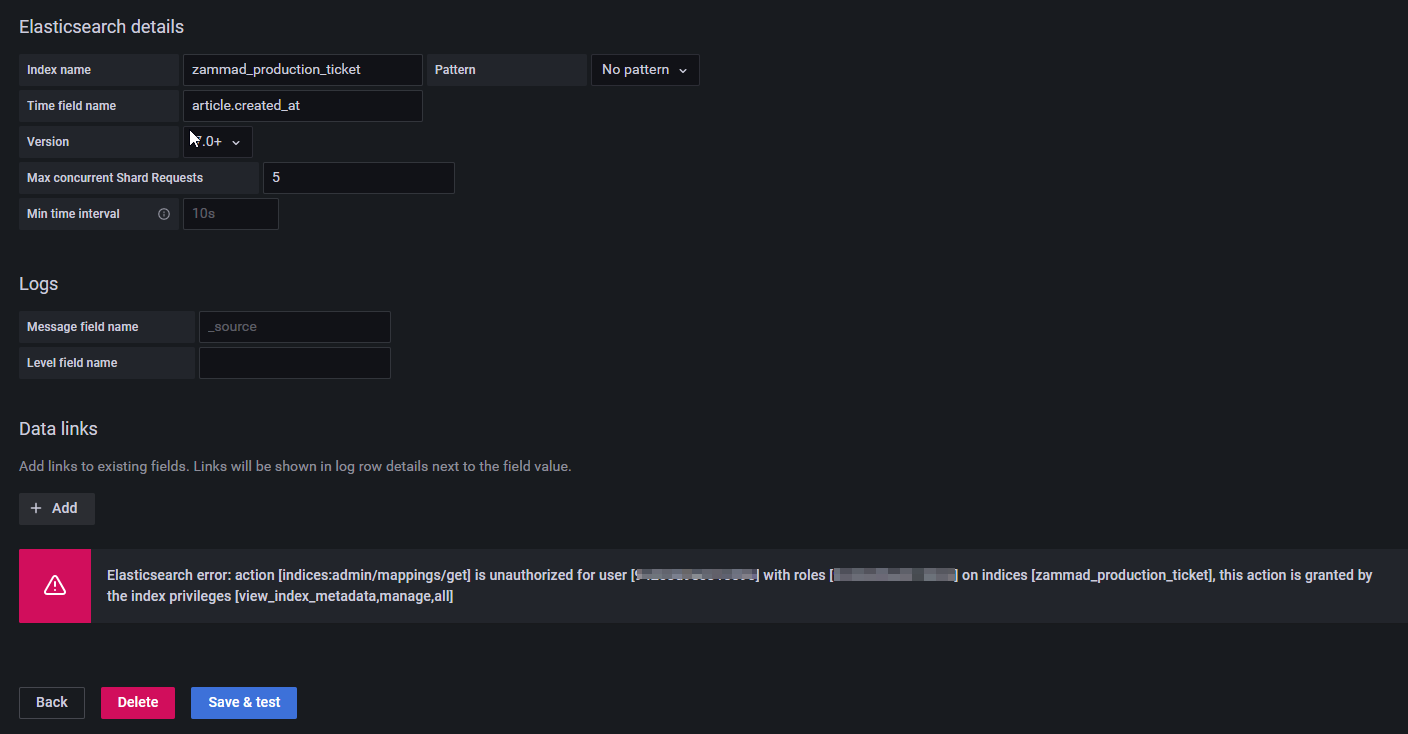The image is a detailed screenshot of an information section related to Elasticsearch. At the top, a prominent title reads "Elasticsearch Details." The remainder of the text is relatively small and challenging to read, but distinct sections labeled "Logs," "Data Links," and another segment that hints at version information are visible. Notably, the version number is partially obscured by the cursor, and an annotation or button labeled "Add One" can be seen.